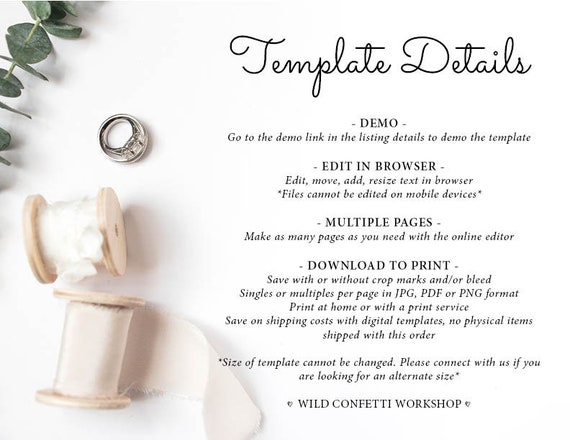The image depicts a white poster designed with an elegant and sophisticated aesthetic. On the top left, there are green vine leaves adding a touch of organic charm. Dominating the center-left is a silver ring, poised above two light cream spools with white ribbons, evoking the feel of a wedding invitation.

However, the text on the right side of the poster reveals it to be an advertisement for a word processing application. The heading, "Template Details," is elegantly written in black script, followed by four main sections of information. These sections include "Demo: Go to the demo link in the listing details to demo the template.", "Edit in Browser: Edit, move, add, resize text in the browser. Files cannot be edited on mobile devices.", "Multiple Pages: Make as many pages as you need with the online editor.", and "Download to Print: Save with or without crop marks and/or bleed. Singles or multiple per page in JPG, PDF, or PNG format. Print at home or with a print service. Save on shipping costs with digital templates. No physical items shipped with this order. Size of template cannot be changed. Please connect with us if you are looking for an alternate size."

At the bottom of the poster is the name of the creator, "Wild Confetti Workshop," rendered in black text, all unified in a stylish, minimalistic composition.